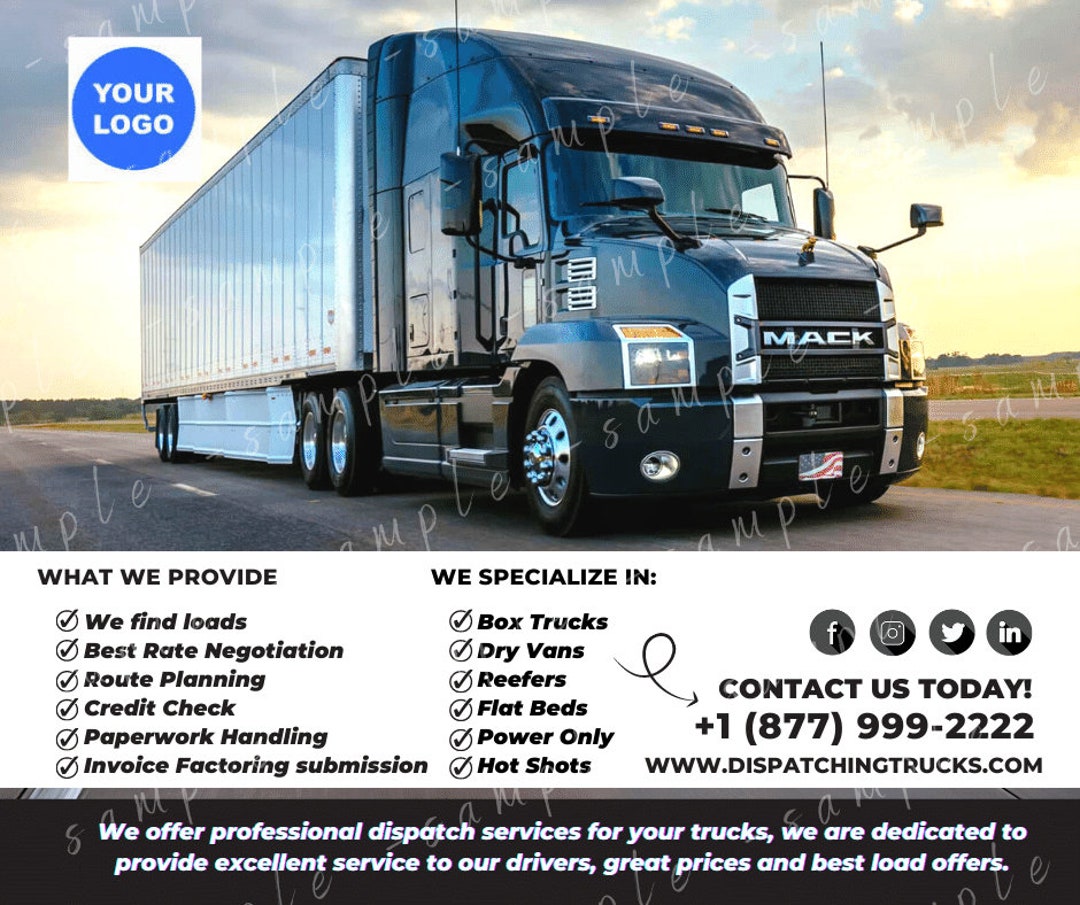This advertisement features a well-composed image and informative text, presenting a compelling offer for professional truck dispatch services. 

At the top of the ad, a striking photograph captures a blue Mack Truck, set against a backdrop of a clear sky and a flat, grassy landscape. The truck, positioned on a road, has a blue cabin and a white cargo area, with five visible tires from the side angle. The cargo area appears to be empty, suggesting the truck is ready for its next haul.

Beneath the image, a white section houses detailed information in organized lists. The first list outlines the services provided, including load finding, best rate negotiation, route planning, credit checks, paperwork handling, invoice factoring, and submission. The second list specifies the types of trucks the service specializes in: box trucks, dry vans, reefers, flatbeds, power only, and hotshots. Social media icons for Facebook, Snapchat, Twitter, and another unspecified platform are also displayed, indicating the company’s online presence.

At the bottom, in a black footer, the contact information is clear: "Contact us today 1-877-999-2222 www.dispatchingtruck.com." The footer also includes a dedication statement to their professional dispatch services, emphasizing their commitment to providing excellent service to drivers, offering great prices, and securing the best load offers.

This detailed and visually appealing advertisement effectively communicates the extensive services and benefits offered to truck drivers.